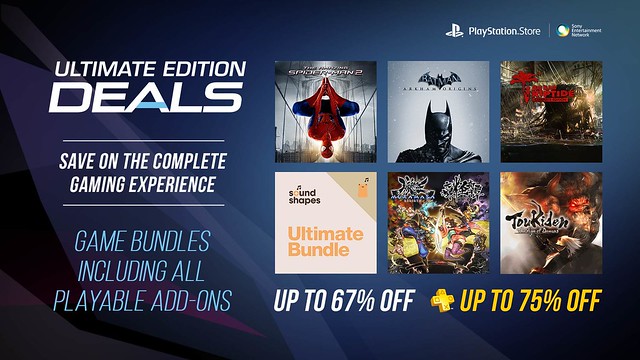Screenshot of the PlayStation Store Website for Ultimate Edition Deals

This is a screenshot of the PlayStation Store website, presumably viewed on a PS4. The top right corner prominently displays the PlayStation Store logo. Adjacent to the logo, the text reads "Sony Computer Entertainment," affirming the platform. On the left side of the screenshot, the featured promotion is for "Ultimate Edition Deals," with the headline styled in a large font, incorporating a blue swish within the letter 'A.' Beneath this headline, the subtext reads, "Save on the complete gaming experience." Further down, additional light blue text highlights "game bundles including all playable add-ons."

On the right side of the screenshot, six game covers are displayed in a 2x3 grid pattern, showcasing the following titles from top left to bottom right:

1. Spider-Man 2 or The Amazing Spider-Man 2
2. Batman: Arkham Origins
3. Dead Island: Riptide
4. Sound Shapes: Ultimate Bundle
5. Unknown title, possibly Muramasa: The D&B (uncertain)
6. Toukiden

At the bottom of the screenshot, there's a promotional banner stating, "Up to 67% off," with an additional offer indicating, "With Plus, you get up to 75% off."

This detailed description provides a comprehensive overview of the screenshot, summarizing its promotional content and layout.